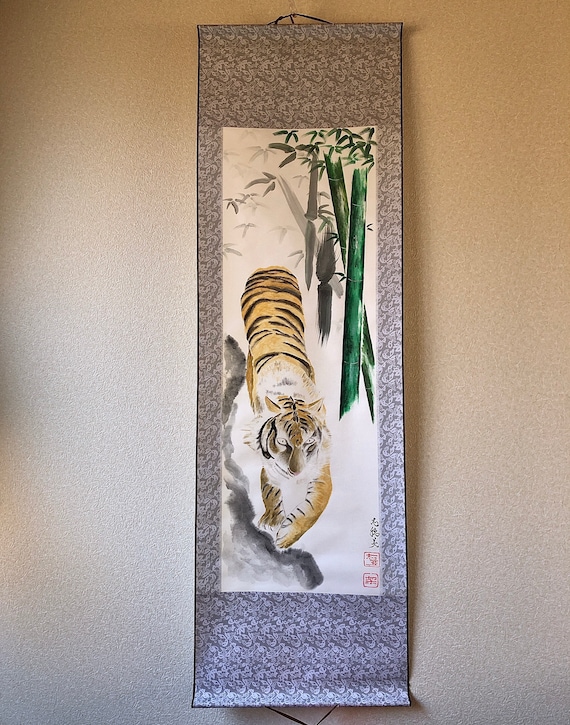This image depicts a detailed wall hanging on a speckled light tan to gray wall. The hanging is a rectangular tapestry with a thin black border adorned in gray and white floral patterns, extending along the top, bottom, and sides. In the center of the tapestry, a vivid scene unfolds on a white background: at the top right corner, green bamboo stalks and leaves gracefully arch towards the top center, subtly transforming into shades of gray. Below, on a gray rock, an orange and black-striped cheetah is meticulously painted, shown from an elevated perspective as it crawls, revealing its detailed front and back legs. The cheetah’s face is distinctly visible with its expressive eyes and ears. In the bottom right corner of this central image, there is elegant Asian script, adding to the cultural essence of the artwork.